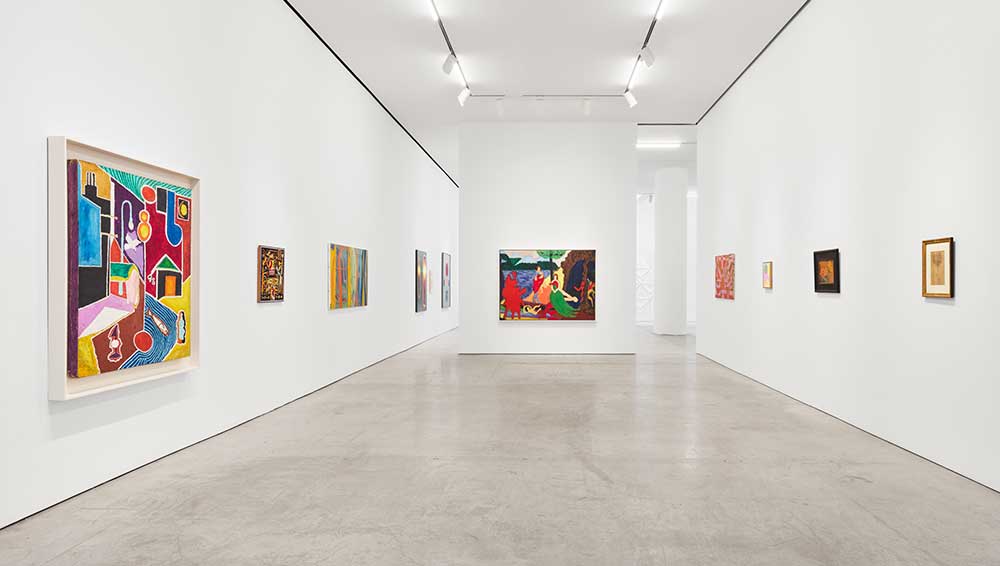The image depicts a large, pristine art gallery room with white walls, a white ceiling, and bright overhead lighting that reflects off the shiny, white-and-gray floor. The space features a central divider wall, creating paths along either side for viewers to appreciate the artwork. On the left-hand side, there are five framed art pieces, including at least two abstract paintings. The right-hand side showcases an additional four framed canvases. The divider wall itself holds a striking painting depicting four women. A fine line runs along the edges of the ceiling and floor, which may be part of the gallery's minimalist design aesthetic. The overall ambiance is one of modern elegance, emphasizing the artwork on display.